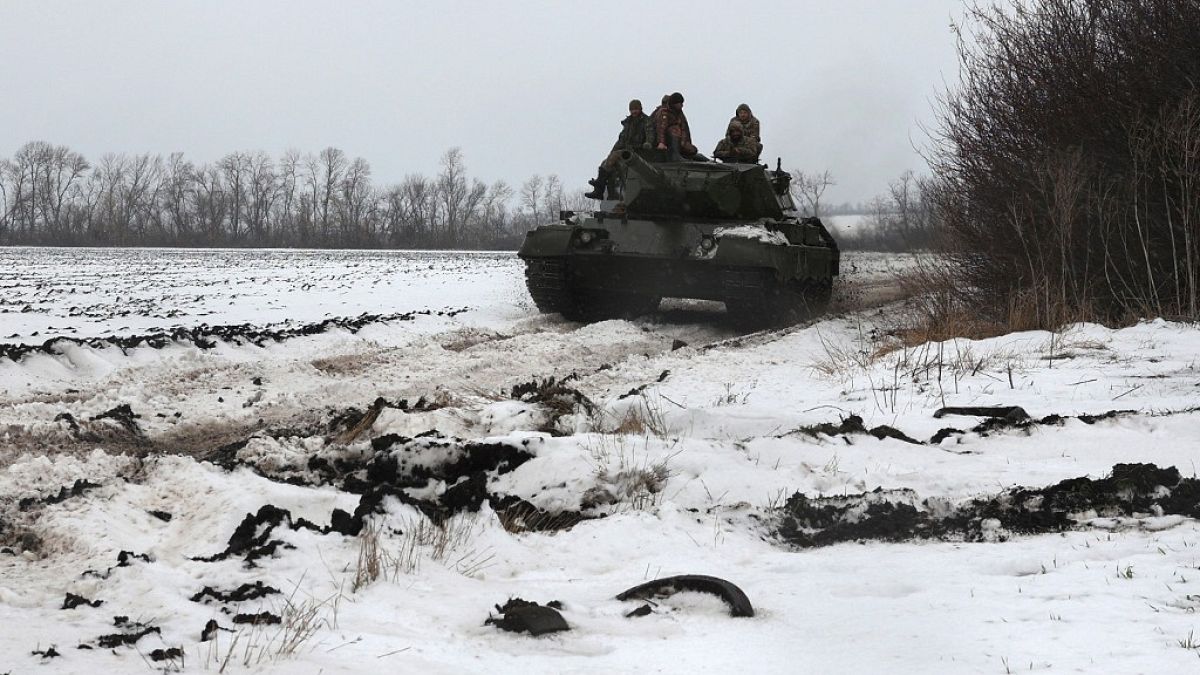In this winter landscape, under an overcast sky tinged with light blue and gray, a dark, possibly green or black tank rumbles forward along a snowy and icy track. The ground is blanketed in snow, creating a stark, desolate scene that is accentuated by the bare, craggy winter trees and dead bushes in the background. The tank, with its commanding presence and large gun barrel, is accompanied by about six soldiers who are perched on top, dressed in winter gear including jackets, hats, and helmets that blend seamlessly with the tank's dark exterior. The flat, open terrain reveals faint indents where other vehicles have passed, indicating a well-trodden path through the desolate wilderness. The soldiers, presumably wearing camouflage patterns, appear vigilant as they navigate this bleak, frosty expanse.